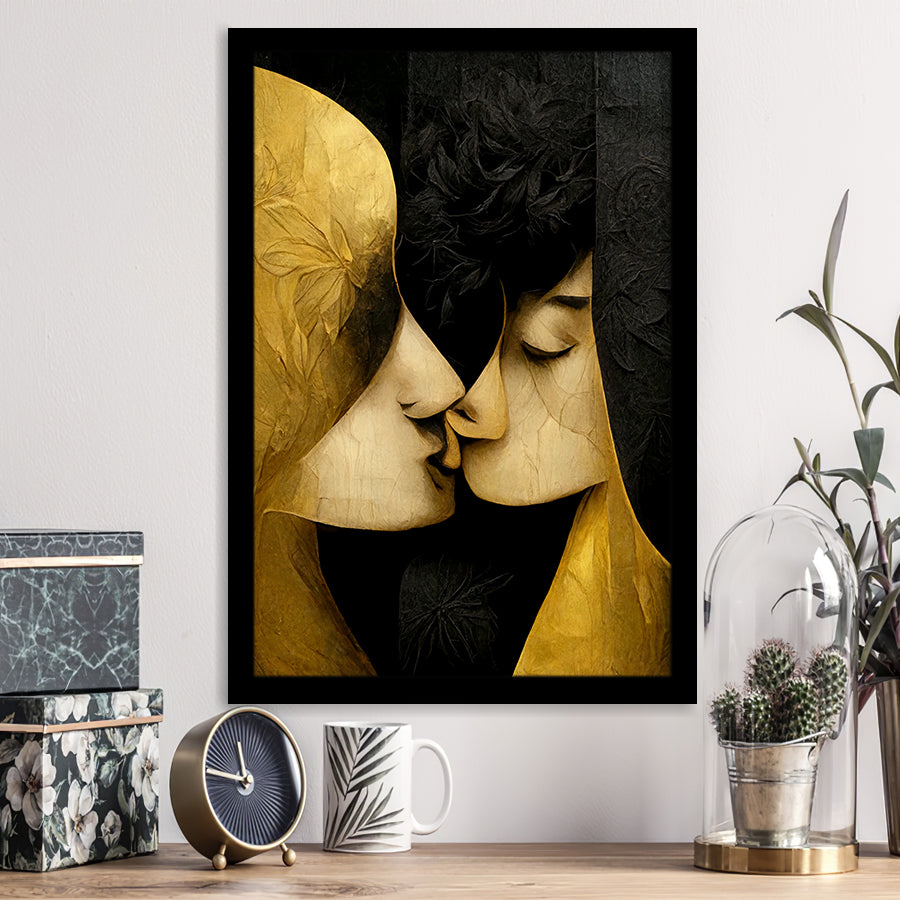The image shows a tasteful and neatly arranged scene inside a house. The wall, painted in a neutral, light beige color, features a large abstract painting of two people kissing. This artwork, framed in black, predominantly uses shades of black, gold, and a yellowy bone color to depict a male and a female, with the female wearing a hat adorned with leaves and the male characterized by long bushy hair, dark eyebrows, and dark eyeshadows. The painting takes up roughly a third of the wall space and hangs about nine inches above a wooden dresser.

Resting on the dresser from left to right are two decorative guest boxes stacked on top of each other. Beside these boxes is a vintage, round clock with a shiny face, gold trim, and a patterned interior, displaying the time as 10 to 12. Next to the clock is a white bone china coffee mug decorated with fern leaf patterns. Moving further right, there is a small cactus housed in a tin bucket, placed inside a bullet-shaped glass terrarium with gold trimming at the base and around the glass frame. Adjacent to the cactus, towards the rear and slightly to the side, sits a vase partially visible and holding a stemmy flower, mostly consisting of leaves. The described arrangement gives the room an elegant yet cozy aesthetic.